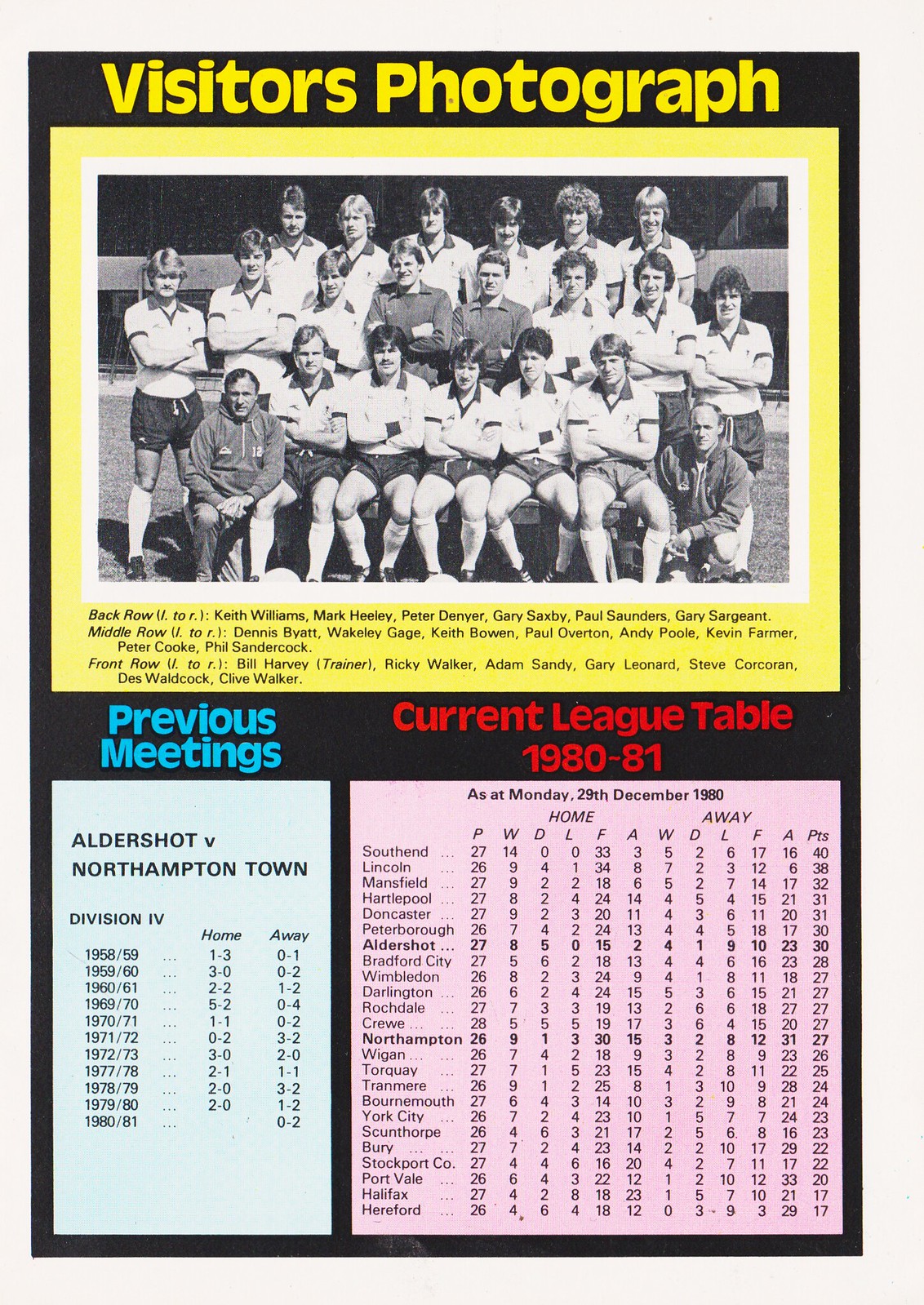The image is a detailed page from a sports magazine showcasing an old soccer team program. At the top, there's a yellow-framed, black-and-white photograph of a soccer team from the 1970s, with the text "Visitors Photograph" above it in yellow. The team is arranged in three rows, with the first row mostly seated or kneeling, likely featuring two coaches on the ends, while the second and third rows are standing. Below the photograph, there's a list of players' names corresponding to their positions in the photo.

On the lower left part of the page, a blue header reads "Previous Meetings," detailing past matchups between Aldershot and Northampton Town in Division 4, with columns showing scores and dates from various home and away games. In the lower right section, a red header says "Current League Table 1980 to 81," followed by details of the league standings as of Monday, December 29th, 1980, presented in a pink square, listing different teams and their statistics. The entire layout is enclosed within a black frame, giving it a cohesive and organized appearance.